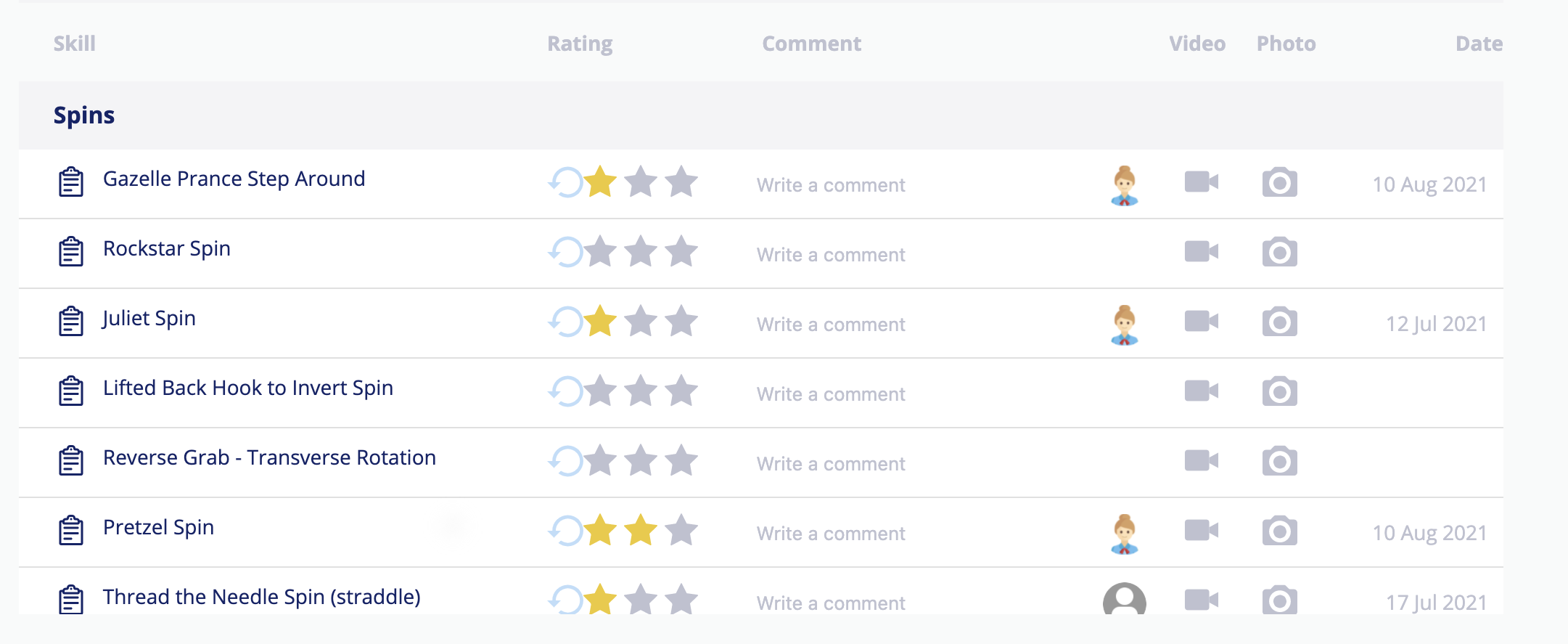**Detailed Image Caption:**

In this screenshot, the interface features a light grey background with multiple navigational tabs positioned at the top of the page. Below the tabs, a structured table is depicted with six columns labeled: "Skill," "Writing," "Comment," "Video," "Photo," and "Date."

- **Skill Column**: This column lists different skills which include:
  1. **Gazelle, Prince, Step Around** - Rated 1 star. Date: August 10, 2021.
  2. **Rockstar Spin** - No rating or date.
  3. **Judo Spin** - Rated 1 star. Date: July 12, 2021.
  4. **Lifted Back, Hover to Invert Spin** - No rating or date.
  5. **Reverse Grab, Transverse Rotation** - No rating or date.
  6. **Puzzle Spin** - Rated 2 stars out of 3. Date: August 10, 2021.
  7. **Thread the Needle Spin** - Rated 1 star. Date: July 17, 2021.

- **Writing Column**: Appears to be unused or empty.

- **Comment Column**: Contains a single text directive: "Write a comment on every skill."

- **Video Column**: Displays a grey icon representing a video camera.

- **Photo Column**: Shows a grey icon of a camera.

- **Date Column**: Lists specific dates next to several skills, corresponding to their entry or rating dates.

The first three skill ratings, described with one star each, have been evaluated by the same user, identifiable by an avatar featuring a blue shirt. The final entry with a rating, "Thread the Needle Spin," was rated by a different user.